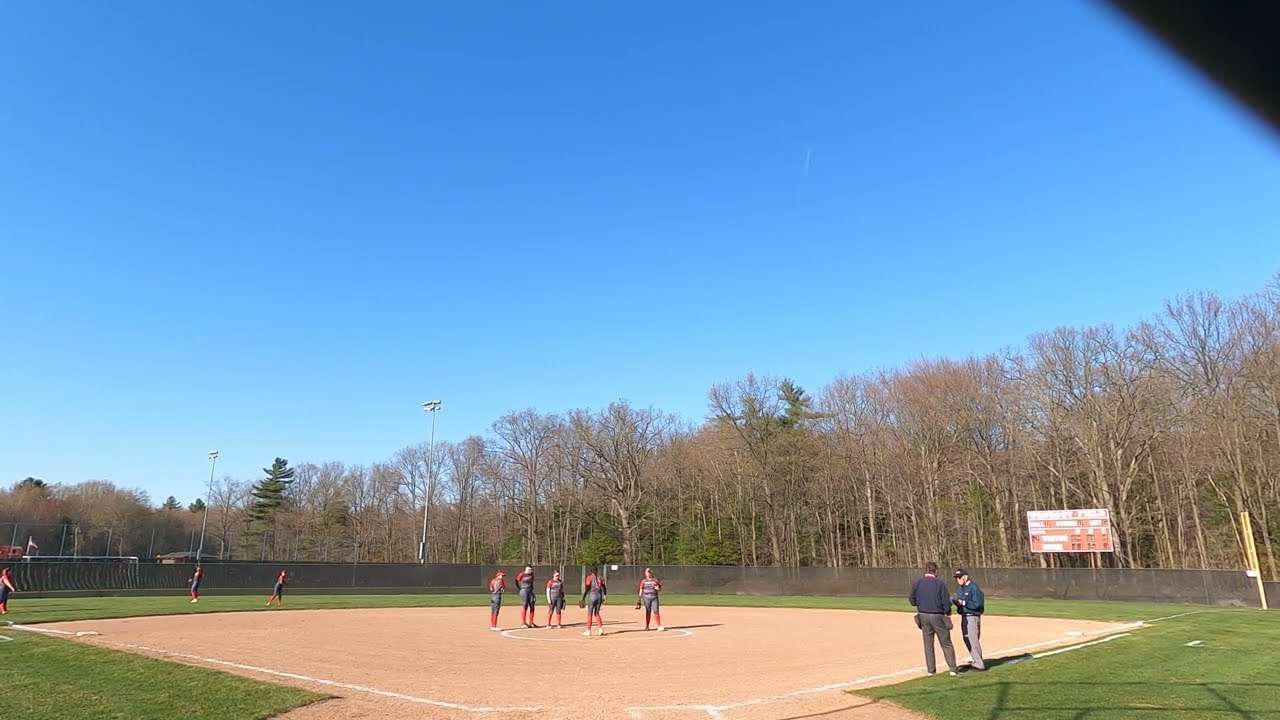The image captures a girls' softball game on a beautifully clear day with a vivid blue sky. Dominating the scene is a meticulously manicured baseball diamond, with bare earth forming the infield and fresh green grass enveloping it. The infielders are clad in gray uniforms accented by strikingly bright red stockings. A group of five players is huddled around the pitcher's mound, perhaps in conversation, while three more players are dispersed in the outfield. Prominently, two men—likely coaches—stand near the first baseline, distinguishable by their lack of uniforms. A scoreboard is visible off to the right, contributing to the organized atmosphere of the field. The entire area is enclosed by a short black chain-link fence, beyond which lie trees that are just beginning to bud, suggesting a spring setting. A serene blue sky overhead ensures that it's a perfect day for softball.